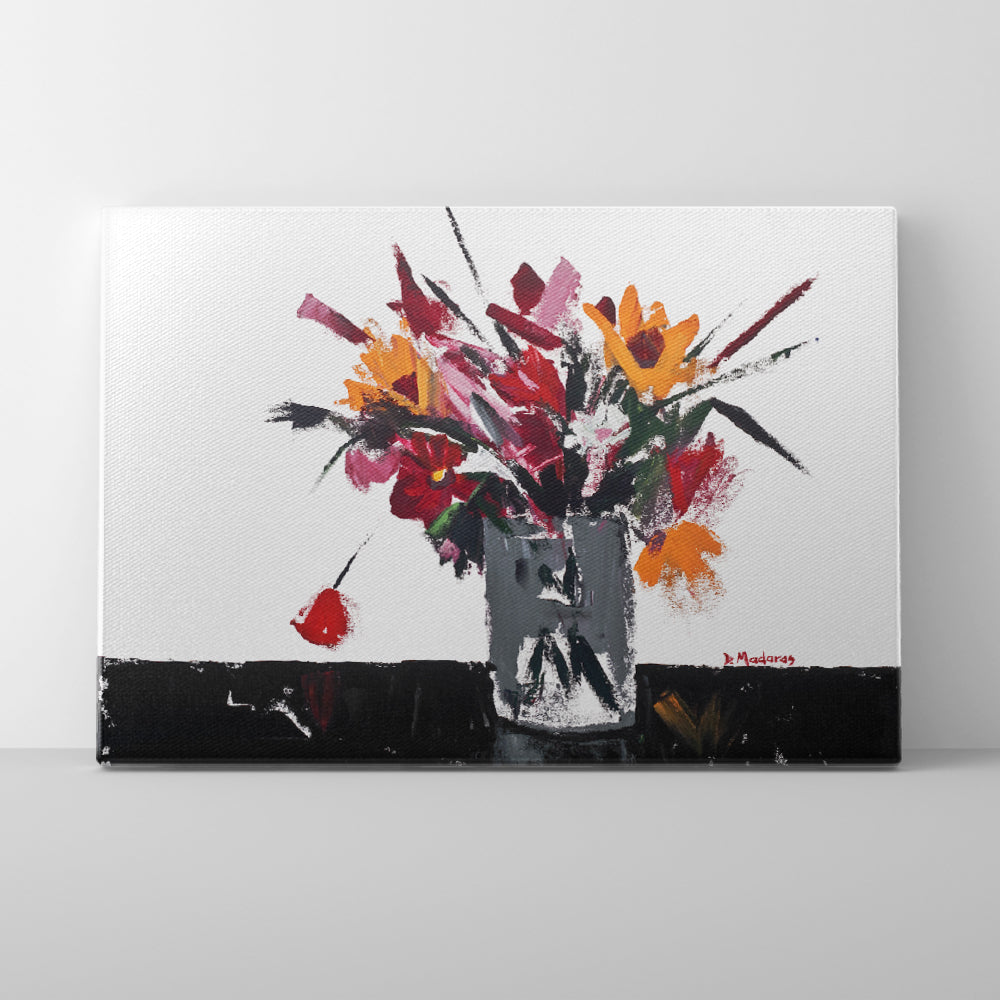The image depicts an advertisement for a painting on a canvas set against a white background. The canvas features a gray base with a vase placed on a nearly solid black surface occupying the bottom portion. Emerging from the vase are flowers painted in vibrant hues of red, orange, pink, and yellow, accentuated by green leaves, crafted with broad, hurried brush strokes that give an impressionistic feel. The stems of the flowers appear in black, contributing to the abstract quality of the piece. A small, red signature reading 'D. Madaris' is noticeably placed on the black surface to the right of the vase, adding a personal touch to the artwork. The painting, resting on a gray surface, juxtaposes the stark white background, making the striking colors of the floral arrangement stand out vividly.